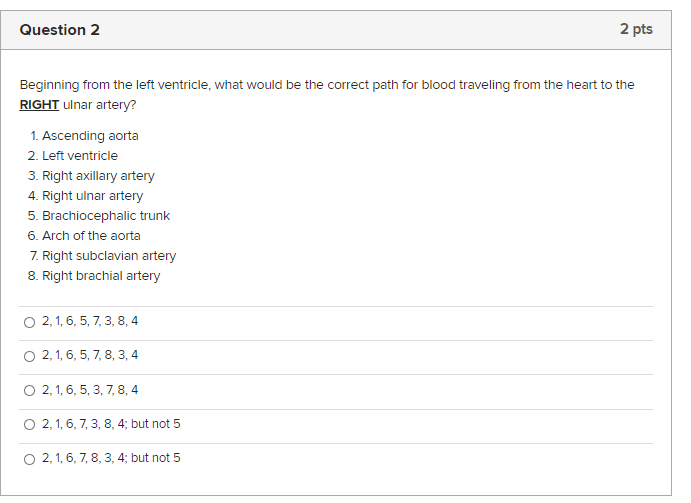The image appears to be a screenshot of a question interface from a digital device, likely a computer or smartphone. The entire layout is encased within a thin black border. At the very top of the image, a light gray strip runs horizontally, displaying the text "Question 2" on the upper left in black font and "2 points" on the upper right. 

Beneath this gray bar, the background shifts to a white color. In slightly less bold black font, the question is presented: "Beginning from the left ventricle, what would be the correct path for blood traveling from the heart to the right **ulnar artery**?" The emphasis on "right ulnar artery" is achieved with bold and underlined formatting.

Following the question, eight potential answers are listed, each prefixed by a small number:
1. Ascending aorta
2. Left ventricle
3. Right axillary artery
4. Right ulnar artery
5. Brachiocephalic trunk
6. Arch of the aorta
7. Right subclavian artery
8. Right brachial artery

A thin gray line separates the question and answer choices. Each choice is accompanied by a small circle, indicating a radio button for selection, all of which are currently unfilled. This layout clearly presents multiple-choice options for the user to click and select the correct path for blood flow from the heart to the specified artery.